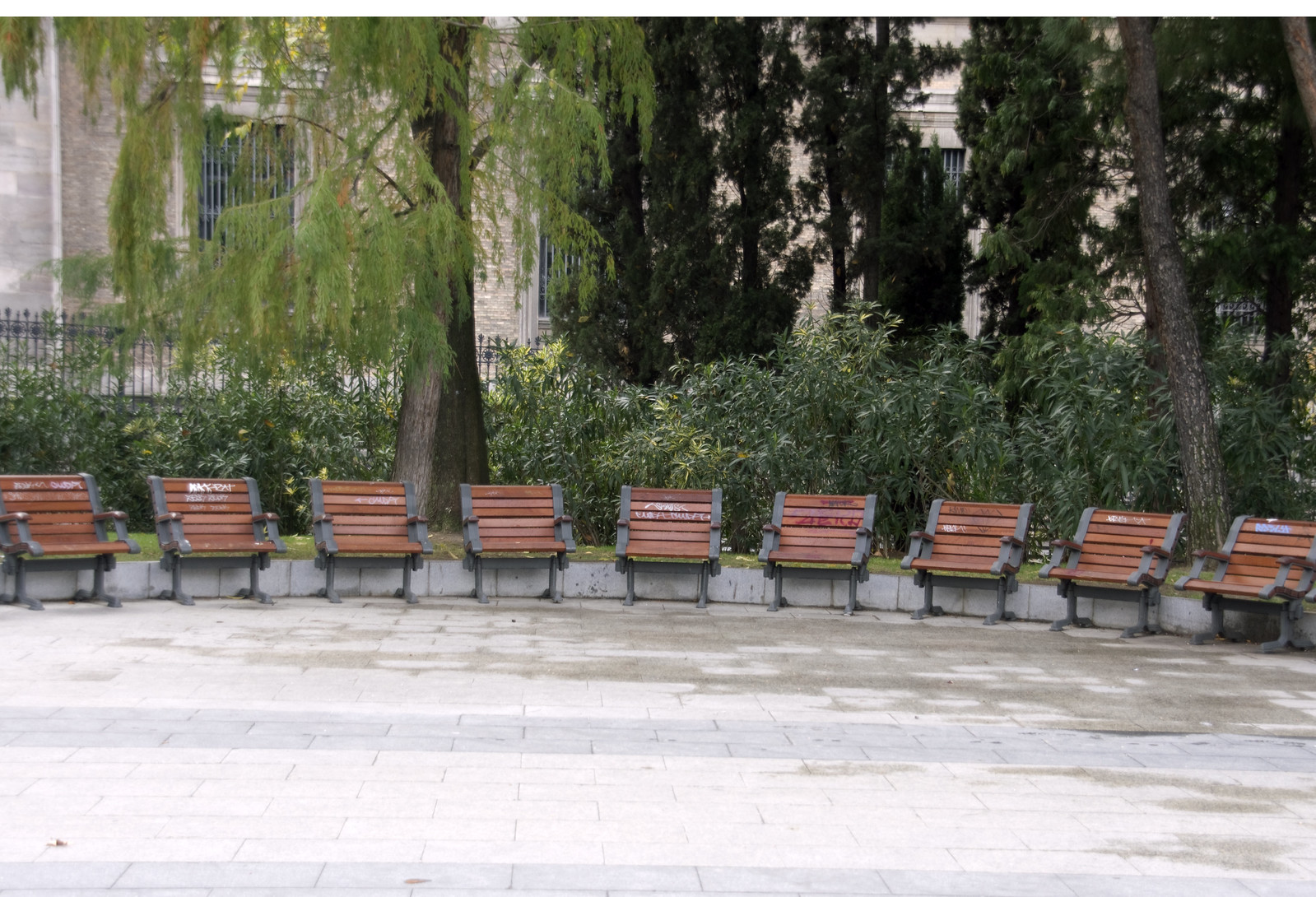The image captures a serene courtyard with a beige stone floor interspersed with strips of darker brown stone. Arranged around the courtyard are numerous wooden benches with short legs, designed to seat one person comfortably or perhaps two children. These benches feature brown armrests and frames that seem to be crafted in a sturdy silver metal or wrought iron. Some benches have visible writing on them in yellow or white lettering, though the text remains unreadable from the image's perspective. The short stone wall behind the benches forms a boundary for the courtyard. Beyond this wall, there is a small grassy area dotted with a few tall trees and encircled by dense bushes. Further in the background, a stone building stands with a metal fence in front of it, adding a structured backdrop to this tranquil, garden-like setting.